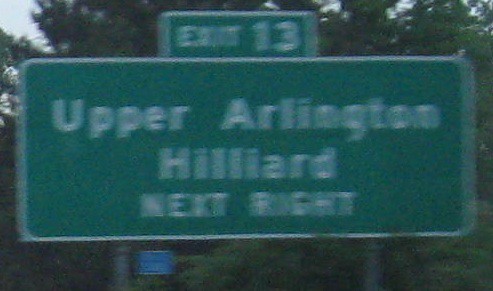This photograph captures a blurry highway sign indicating an exit for Upper Arlington and Hilliard, both suburbs of Columbus, Ohio. The green sign, with its white lettering, reads "Upper Arlington Hilliard, Next Right, Exit 13." Behind the sign, there are trees with lush foliage, suggesting that the photo was taken during the spring or summer.